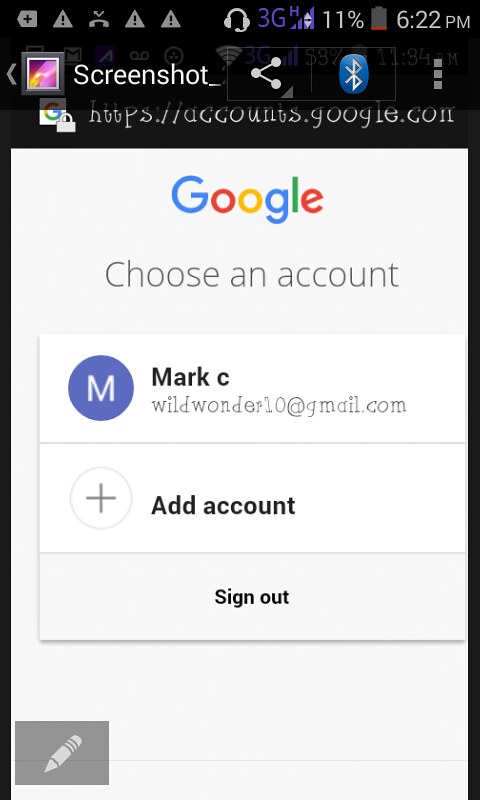This screenshot, captured on a cell phone with a black border, displays the various status symbols typical of a smartphone, including a 3G connection, a battery at 11%, and the time, which is 6:22 PM. The title of the image is indicated as "screenshot," visible at the very top. Noticeable is a prominent Bluetooth icon. The main content of the screenshot is a login page for Google accounts (googleaccounts.com). The header "Google" is clearly visible, adorned in the familiar Google colors of blue, red, yellow, blue, green, and red.

Below the "Choose an account" prompt, only one account is listed: Mark C. His profile icon is a simple purple circle with a white "M" inside, as no photo has been provided. His email address, wildwonder10@gmail.com, is displayed in a cartoonish font. Below his account, there is a white circular button with a "+" sign to add another account, and further down, an option to sign out is provided.

In the bottom left corner, there is a light gray pencil icon inside a dark gray rectangle, which likely provides an option to edit or annotate the screenshot.